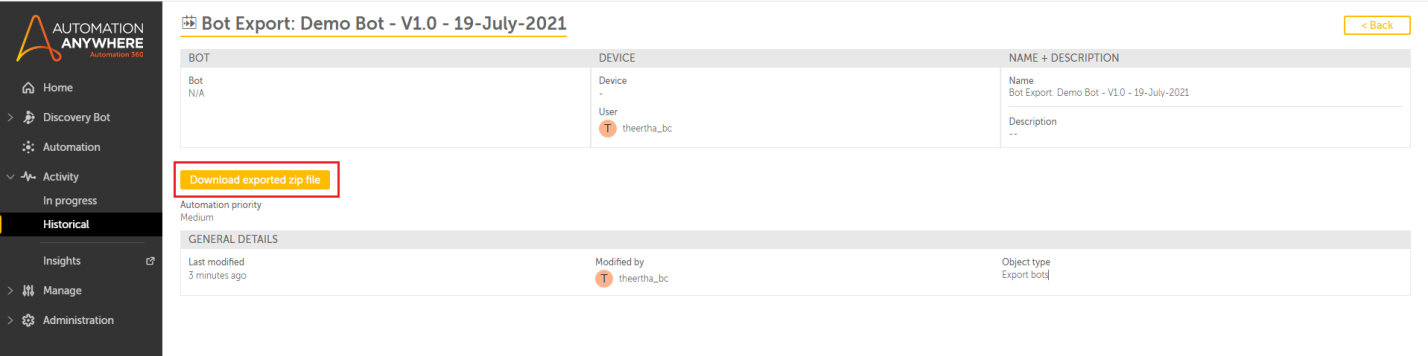This is a detailed screenshot of a web page interface for Automation Anywhere. On the left side, there is a small, vertically-oriented black rectangular box with a list. At the very top-left of this box, there is a symbol resembling a capital letter "A," followed by the text "AUTOMATION ANYWHERE" in capital letters. Below this, "Automation 360" is written in orange. The list includes various categories and subcategories, each with icons beside some of them:

1. Home
2. Discovery Bot
3. Automation
4. Activity
   - In Progress
   - Historical
   - Insights
5. Manage
6. Administration

The right side of the screen, occupying the majority of the space, is divided into two main sections. 

The top section is titled "Bot Export: DemoBot-v1.0-19-July-2021." Below this title, there are several category boxes listed:

- Bot: Under this, it includes "Bots / A."
- Device: This features a user indicated by an icon, which is a pink circle with the letter "T." The username is "THEERTA_BC."
- Next to "Name + Description," it lists:
  - Name: Bot Export, DemoBot, and the date July 21, 2021.
  - Description: (details were not included in the voice note, assumed to be present)

The bottom section of the right side highlights a distinct, clickable bar labeled "Download Export Zip File," which has a yellow background and is outlined in red. Following this section, additional categories are listed:

- Automation Priority: Indicated as Medium.
- General Details:
  - Last Modified: Three minutes ago.
  - Modified by: The symbolic "T" and the user "Theerta BC."
  - Object Type: Export Bots.

This intricate description of the screenshot paints a comprehensive picture of the web page's layout and contents.